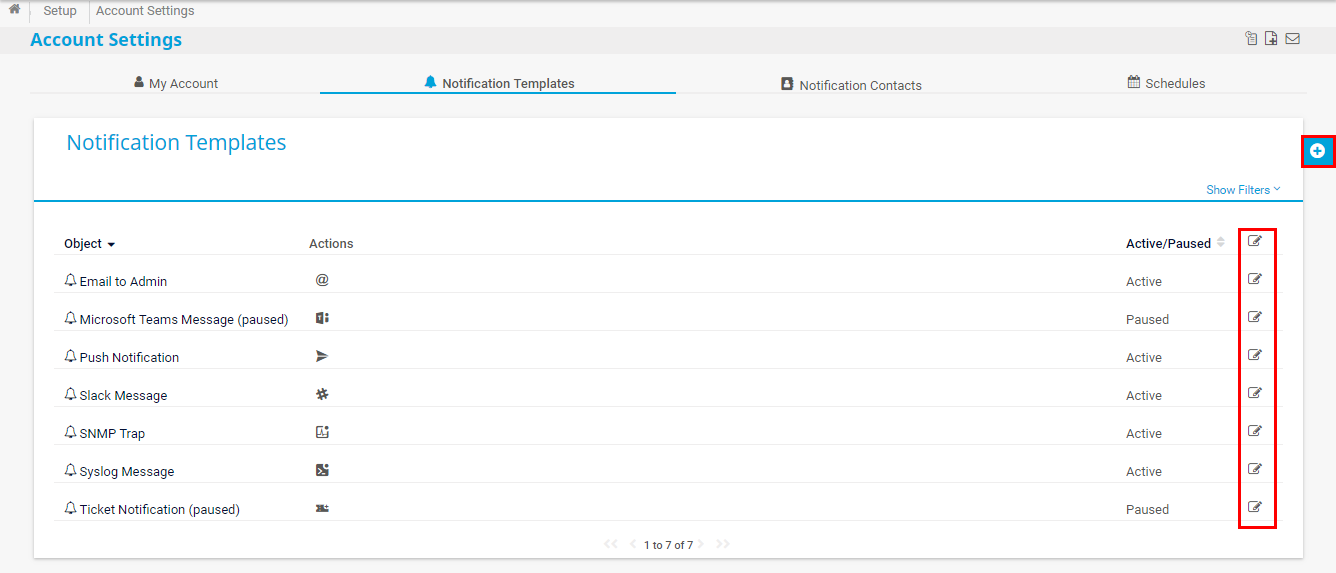Screenshot of a computer screen displaying a web-based organization tool with a white background and a detailed chart. At the top, there are four options labeled in bold letters: "My Account," "Notification Templates," "Notification Contacts," and "Schedules." Below these tabs runs a blue dividing line. Down the left-hand column, various notification channels are listed, including "Email to Admin," "Microsoft Team Messages," "Push Notifications," "Start Message," "SMMT Trap," "Sync Messages," "Ticket Notifications," and "Paused." Adjacent to these entries, checkboxes indicate the status of each function, labeled as either "Active" or "Paused." This interface appears to be an account settings section specifically for managing email distribution and other notification methods.